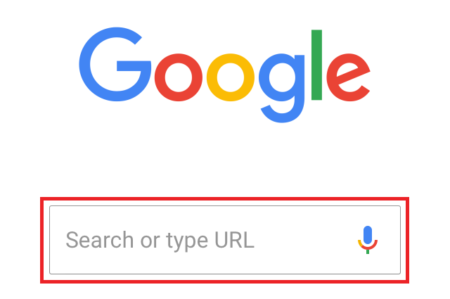The image showcases a portion of a Google search page. Dominating the center is the iconic "Google" logo, prominently displayed in its customary vibrant colors. The logo begins with a blue 'G', followed by a red 'o', a yellow 'o', a blue 'g', a green 'l', and terminates with a red 'e'. Thus, both blue and red appear twice, while yellow and green appear once each. Below the logo, there is a vast expanse of white space. Underneath this white space, there is a rectangular search box with a thin gray border. Inside this search box, the prompt "Search or type URL" is visible. Adjacent to this text is a blue microphone icon, symbolizing Google's voice search feature. Additionally, a subtle gradient of rainbow colors lines the bottom of the microphone icon, adding a touch of color.